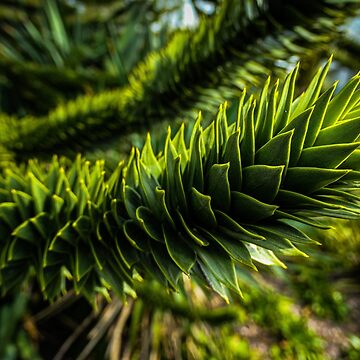This detailed, close-up photograph captures a vibrant green branch of an Araucaria araucana, also known as a monkey puzzle tree. The main branch, prominently positioned, starts near the center-left and gracefully extends upwards towards the top right corner of the frame. Each needle-like leaf, dense and curled, displays a bright green hue with light green edges, tinged almost yellow. The tips of these spiky leaves flare out next to each other and curve upwards. Lit by overhead sunlight, many tips are highlighted, creating a striking contrast with the darker interior. In the soft-focused background, another similar branch reaches upwards unsteadily, reinforcing the main plant's 3-dimensionality and adding depth to the composition. A portion of the clear blue sky is visible in the upper right corner, hinting at pleasant, sunny weather. The image provides an intimate view of the plant's intricate structure, devoid of any other plants or animals, emphasizing the unique beauty of the monkey puzzle tree.